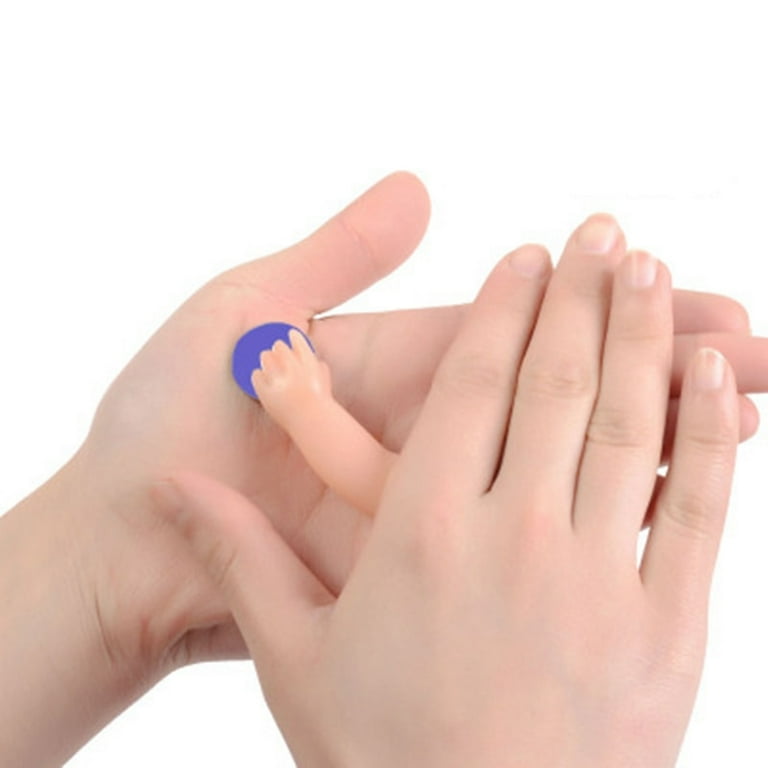The image captures a product photo set against a stark white background, featuring two adult hands positioned together with a small plastic doll hand nestled between them. The left hand appears with its palm facing upwards in a horizontal orientation, while the right hand is nearly perpendicular, with its fingertips resting on the fingers of the left hand and the thumb sticking out. A realistic-looking toy baby hand, extending from a small plastic arm, rests on the left palm and appears to be reaching towards a blue circle. The adult hands, meticulously arranged, create a striking contrast against the white backdrop, drawing attention to the tiny, detailed doll hand and its gesture.